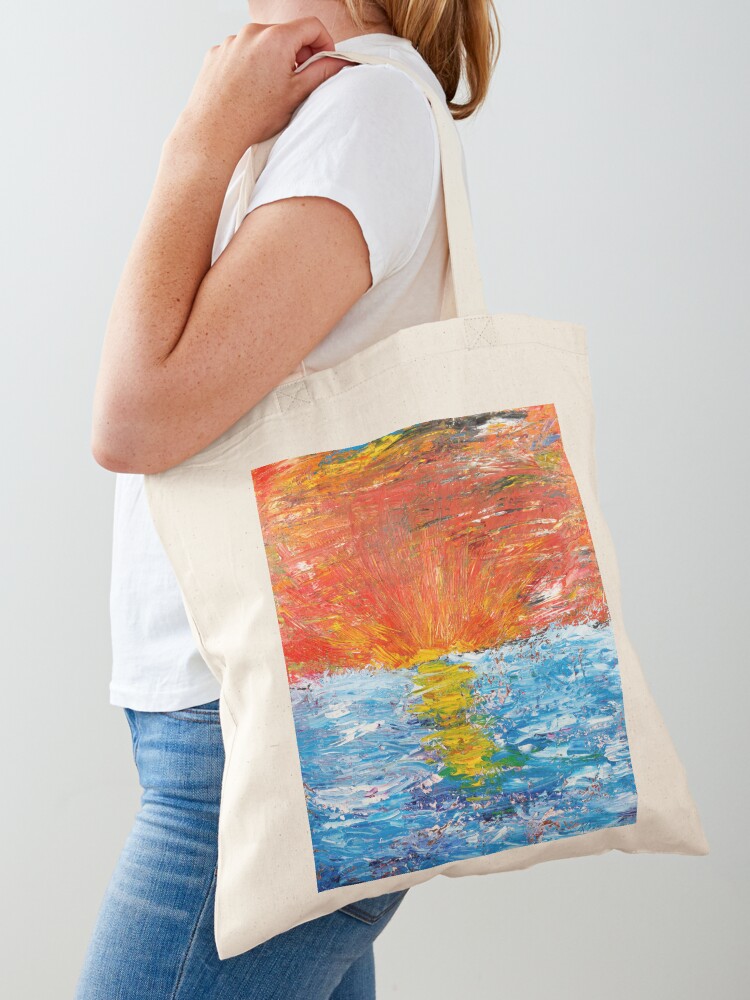The image features a woman with partially visible brown hair, dressed in blue jeans and a white short-sleeved T-shirt. She is modeling a beige tote bag on her left shoulder. The tote bag showcases a distinct, abstract art design. The artwork on the bag comprises a blue lower half with hints of yellow, suggesting a water body, and an orange upper half with touches of yellow, evoking an impression of vibrant, fiery elements. The art is screen-printed, with a sponge-art effect, depicting a mix of circles that could be interpreted as a dynamic and colorful scene. The woman, appearing to be in profile, stands against a plain, possibly gray background in a vertically oriented photograph. The emphasis is on displaying the tote bag as the key subject of the image.